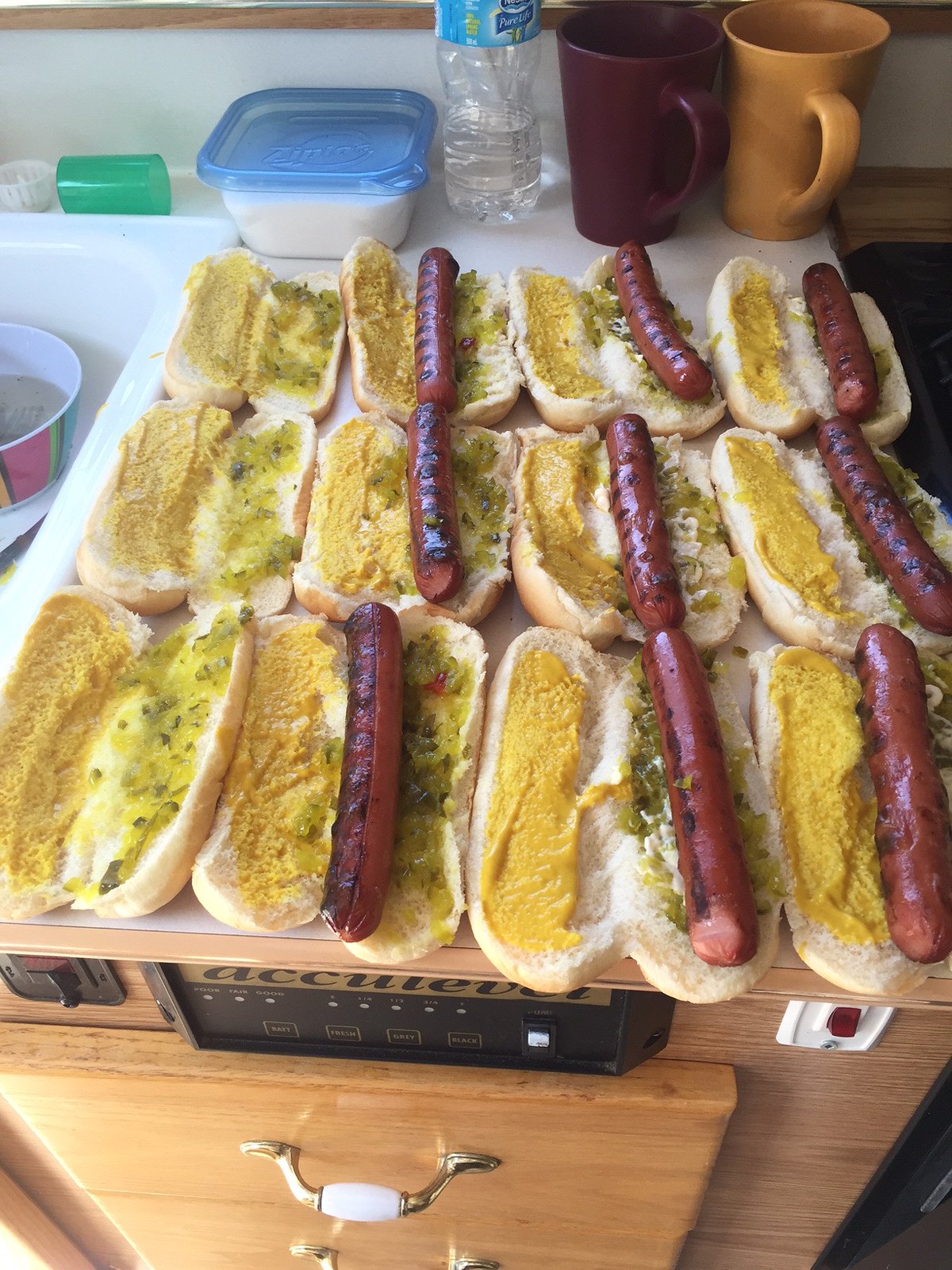This image captures a close-up view of a kitchen countertop where food is being prepared. Spread out in three rows of four, we see a total of twelve hot dog buns. Most of these buns contain grilled hot dogs, identifiable by their grill lines, and all are generously garnished with mustard and green relish. The hot dogs are laid in a pattern where three buns at the beginning of each row remain without hot dogs. Above the buns, the countertop holds a distinctive dark red mug and a mustard yellow mug, along with a partially empty water bottle and a small plastic container, possibly containing sugar or salt. The countertop is positioned next to a sink filled with dirty dishes on the left, and beneath the counter, light wood-grain drawers with brass handles are visible.